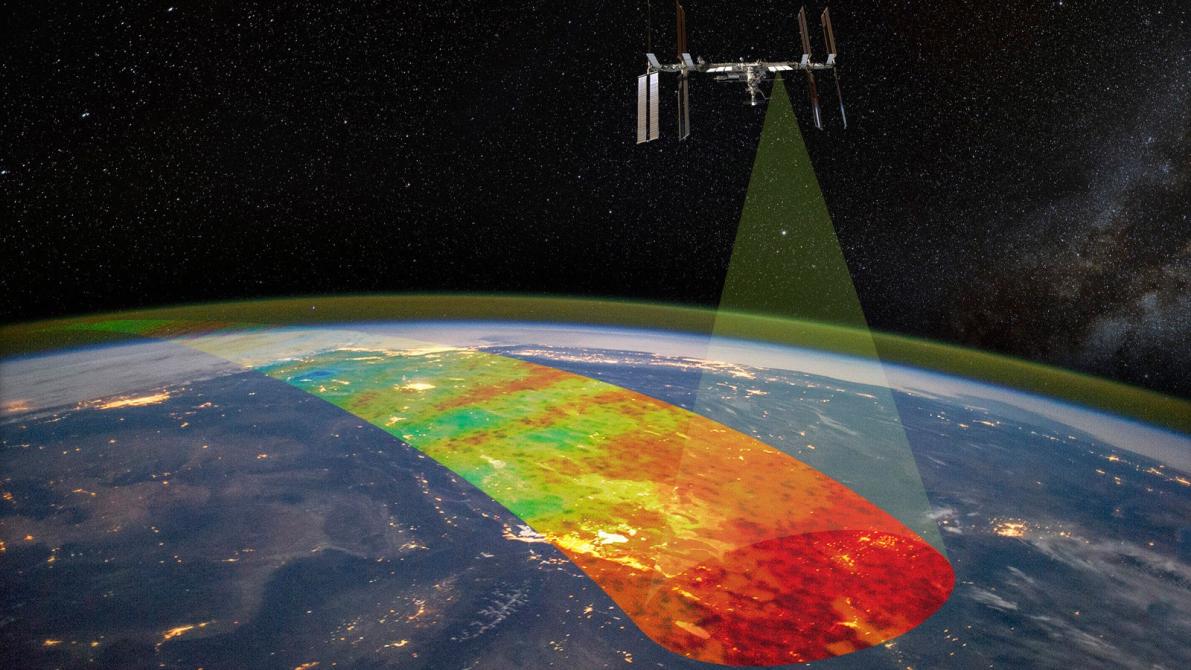The image is an ethereal and vividly colorful representation that appears to portray a scene from outer space, possibly created as digital art rather than an actual photograph. A silver, metallic spacecraft or satellite hovers in the upper part of the image, emitting a golden triangular beam that illuminates a section of the earth below. This light creates a gradient effect on the planet's surface, transitioning from fiery oranges and yellows to serene blues and greens. The earth's curvature is visible, mostly adorned in blue with some green patches. The background is a deep, star-filled black sky, scattered with celestial bodies and planets, enhancing the intergalactic feel. The image lacks textual elements and detailed contextual information but could be reminiscent of illustrations found in science textbooks or on technological and scientific websites. The overall aesthetic suggests a digitally crafted or software-generated artwork.